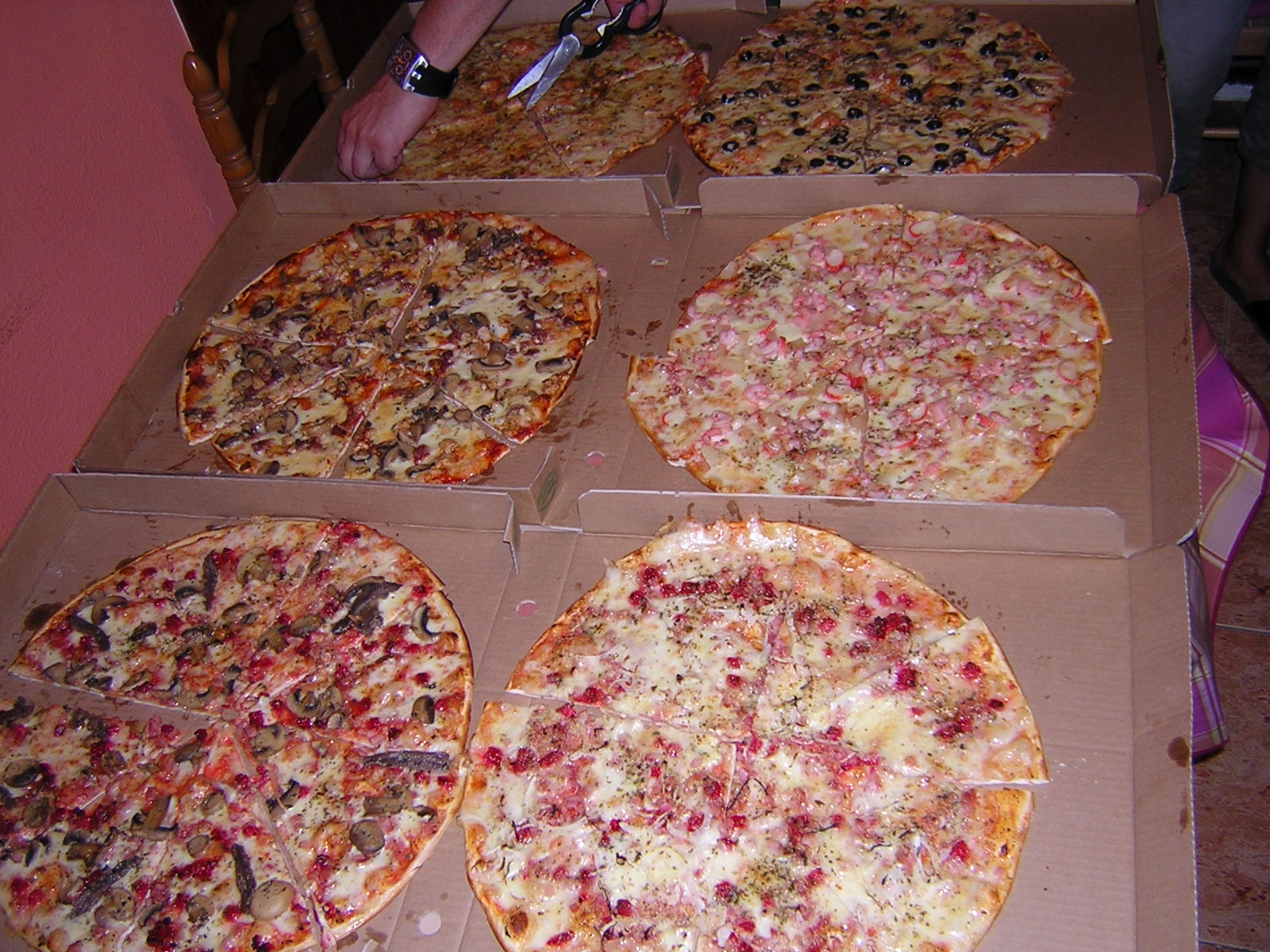The image showcases a scene dominated by six large, thin-crust pizzas, each nestled in open cardboard boxes on a table almost completely obscured by the boxes. Every pizza has distinct toppings, featuring supreme combinations, anchovies, ham and pineapple, mushrooms, Canadian bacon, cheese, seasonings, and black olives. The pizzas are fully intact, suggesting they have not yet been served or eaten. A male Caucasian hand, adorned with a wristwatch, holds a pair of food scissors poised to cut one of the pizzas. The setting is implied to be casual, possibly a party or a restaurant, with a pink or salmon-colored wall in the background. Additional details include a purple checkered tablecloth partially visible beneath the pizzas, a wooden chair on the left, and an overall impression that the pizzas cover about 80% of the photo.